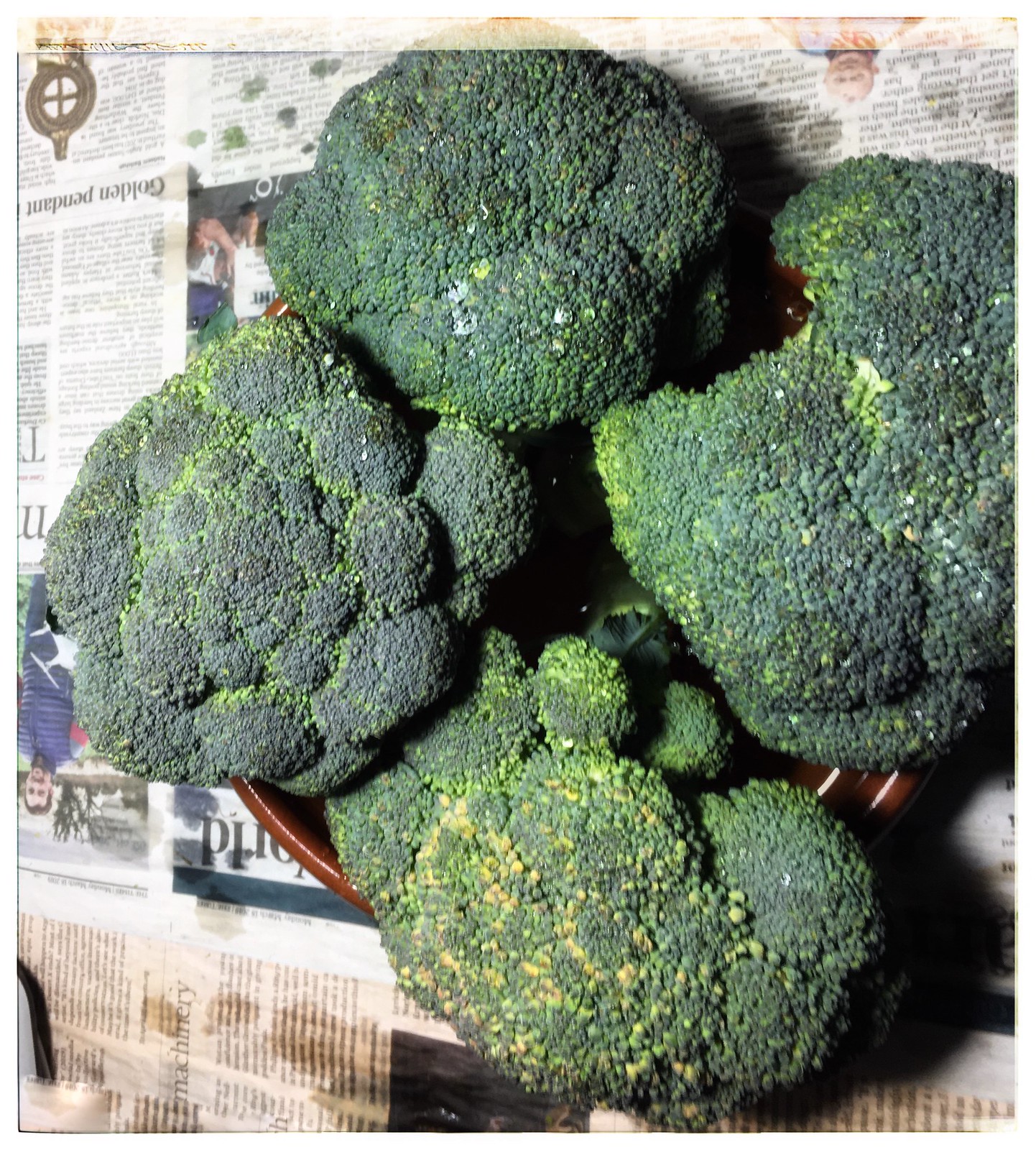In this detailed image, we see a worn, dirty newspaper spread out on a flat surface, marred with various stains including coffee, green, and dirt-like smudges. On top of this newspaper, there is a dark brown bowl, which could be made of plastic or wood. Inside this bowl, there are four large stalks of broccoli. The broccoli is mostly dark green but shows signs of aging, with some yellowing starting to appear, indicating that it is beginning to go bad. Despite the slight discoloration, the broccoli still looks edible. There appears to be a bit of water at the bottom of the bowl, in which the broccoli is sitting. The overall appearance is somewhat nasty due to the filthy newspaper and the aging broccoli.